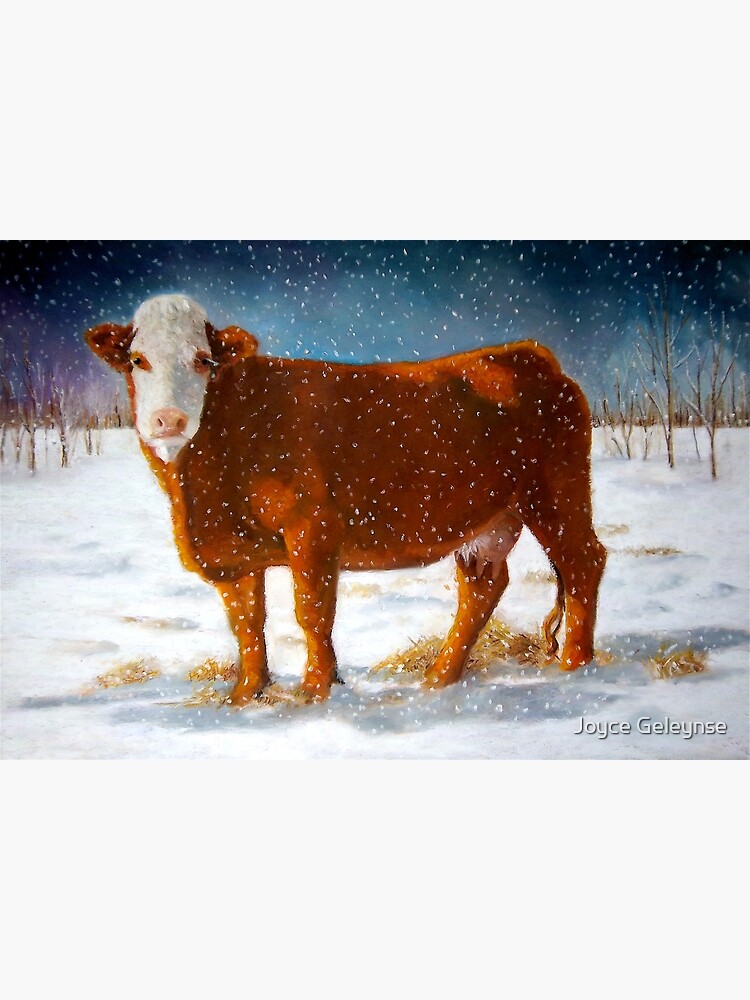This painting, created by the artist Joyce Geleynse, depicts a large cow standing stoically in a snowy landscape. The viewer sees the side view of the cow, which has a dark red-brown body and a distinct white face. The cow is staring forward, directly at the viewer. Patches of brown grass peek through the snow-covered ground, adding texture to the scene. The background showcases a line of dry trees against a sky that is a blend of blue and white, dotted with falling snowflakes. This suggests that it is snowing within the scene. Two light gray horizontal strips frame the top and bottom of the painting, adding a subtle border to the artwork. Additionally, the bottom right corner bears the artist’s name, "Joyce Geleynse," written in white.